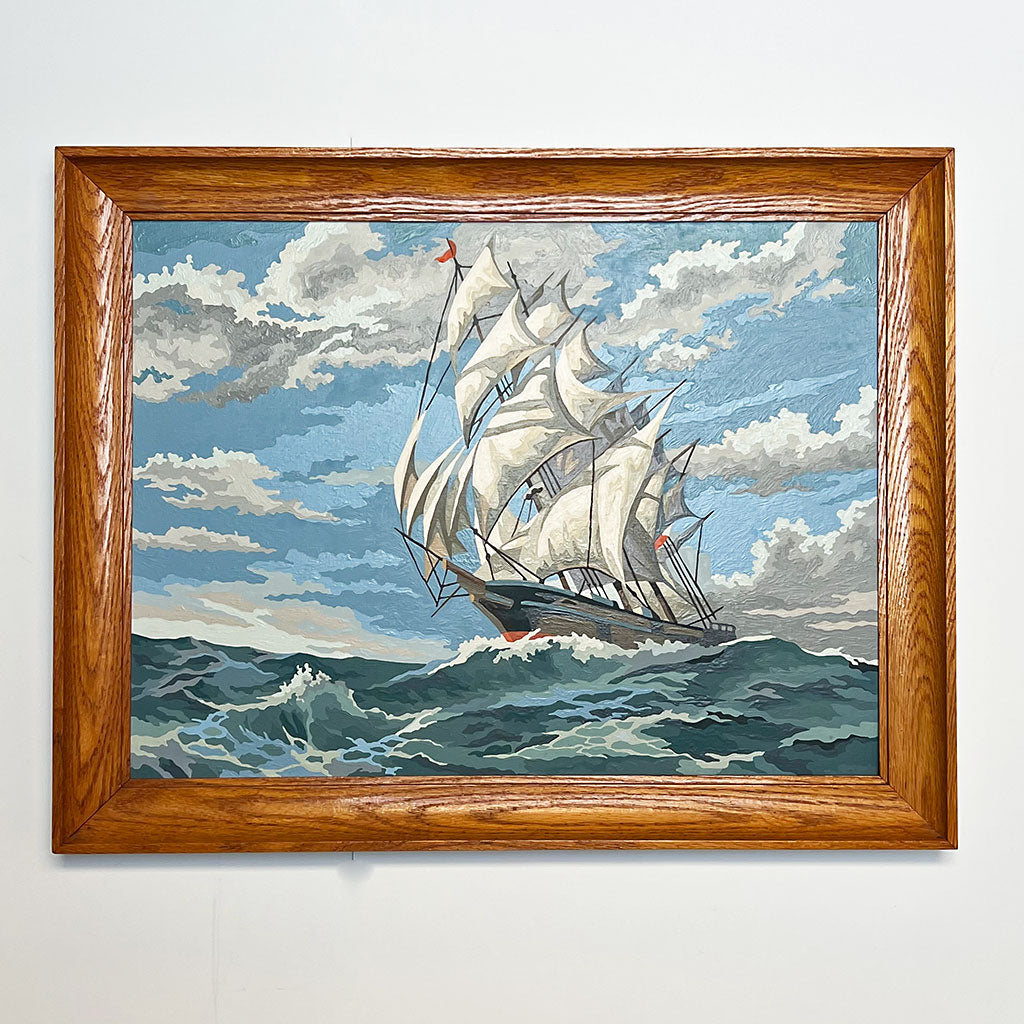The image depicts a painting of a sailing ship navigating slightly rough waters, displayed within a wooden picture frame. The dark wood frame with noticeable grains contrasts against a solid gray background. The ship, facing left, boasts three main masts with numerous white sails of varying sizes, the largest on the tallest mast. The vessel appears to be leaning slightly to its starboard side. The ship's hull is orange at the bottom, transitioning to a dark wood color at the sides. Amidst the choppy waves—highlighted by cresting wave caps—the sea alternates between light and dark shades of blue. Overhead, the sky is a mix of vibrant blue with white, puffy clouds, tinged gray in the top left and bottom right corners. A small red flag adorns the tallest mast, adding a touch of color to the otherwise dramatic maritime scene.